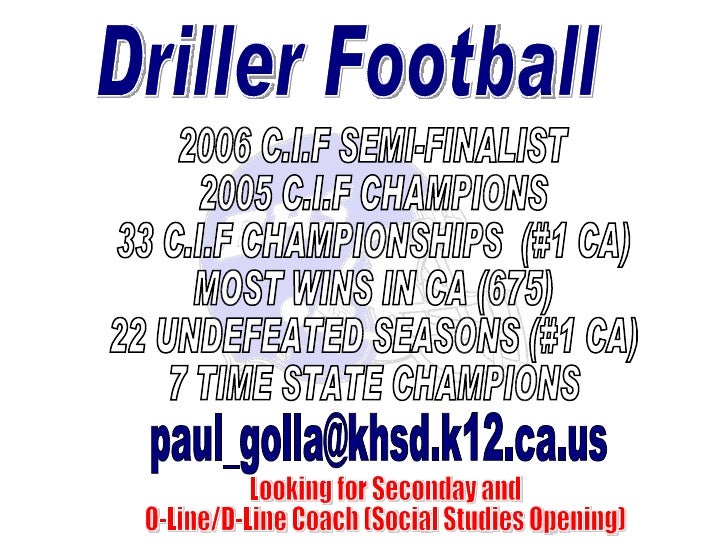The image is a digital advertisement or Facebook post for Driller Football. At the top, in blue letters with a white outline, it proudly announces "Driller Football." Below this, in white letters with a black outline, the accolades of the team are displayed: "2006 CIF Semi-Finalists, 2005 CIF Champions, 33 CIF Championships, Number One in CA, Most Wins in CA (675), 22 Undefeated Seasons, Number One in CA, Seven Times State Champions." Beneath these accomplishments, in blue text, there is an email address: "paul_gola@khsd.k12.ca.us." The poster also features a call for job applicants in red text with a white outline, stating: "Looking for a Secondary and a Zero Line/D Line Coach - Social Studies Ongoing." Backgrounding the text is a faded clipart-style blue football helmet, which appears to have "BRS" or a similar text on it, though it's somewhat obscured by the text overlay.